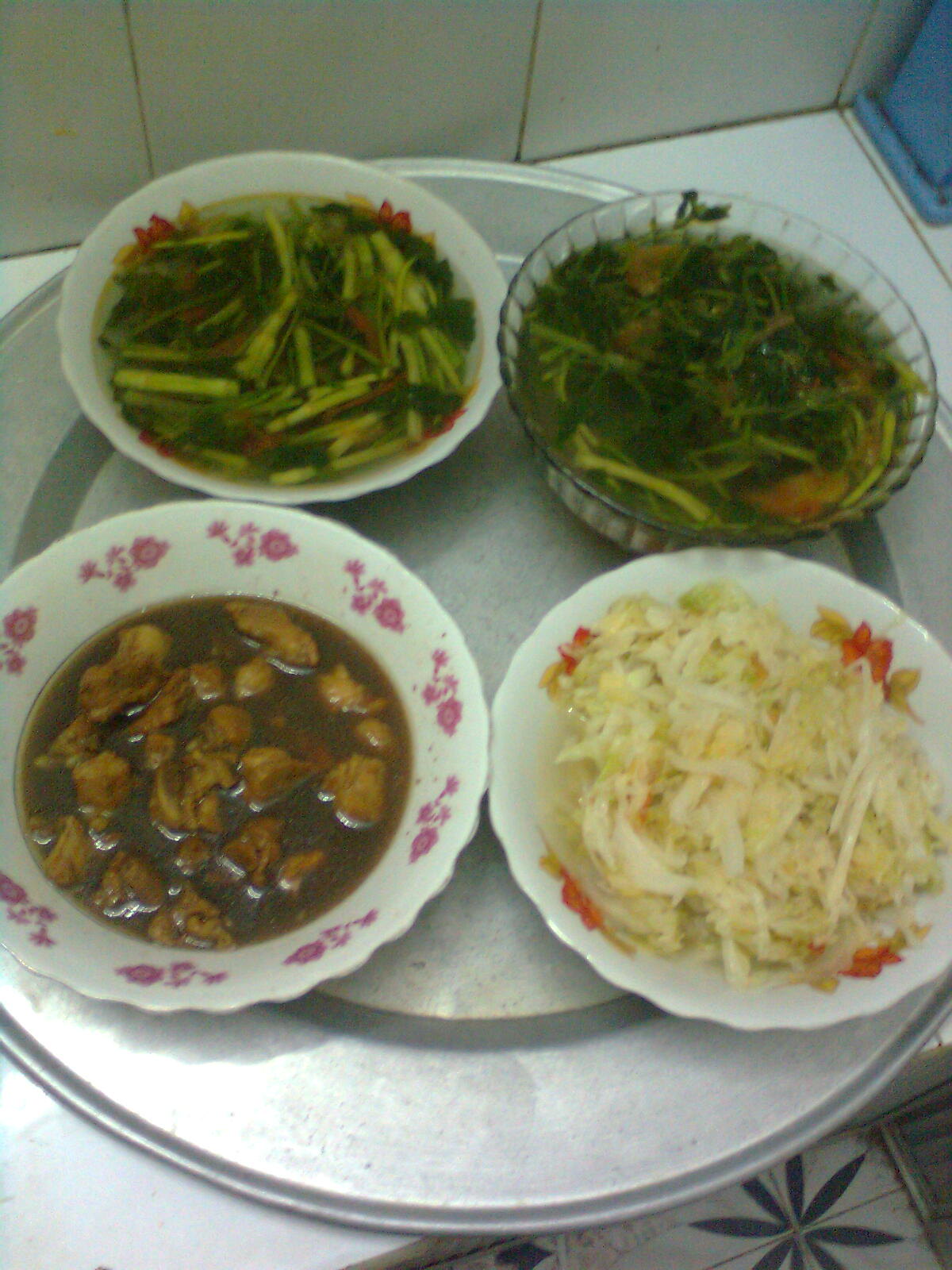The image is a realistic vertical photograph set against a backdrop of what appears to be an off-white tiled kitchen wall with dark brown grout in the top left corner. The bottom right part of the image features a floor with white tiles decorated with a green floral pattern. In the center of the image, a stainless steel serving plate holds four distinct bowls. 

The upper left bowl is white and contains various shades of green vegetables, possibly green beans or similar slender vegetables. To its right, a transparent bowl holds a mix of lighter and darker green vegetables, along with some carrots. In the bottom left, there is another white bowl adorned with pink flowers around the edge, filled with a brown broth that includes pieces of meat, likely chicken, or mushrooms. The final bowl on the bottom right is white and appears to contain a lighter food item, possibly rice or yellow noodles, along with a bit of broth and some white meat.

The photograph seems to capture a moment, possibly in a restaurant, showcasing a neatly arranged meal ready for serving.